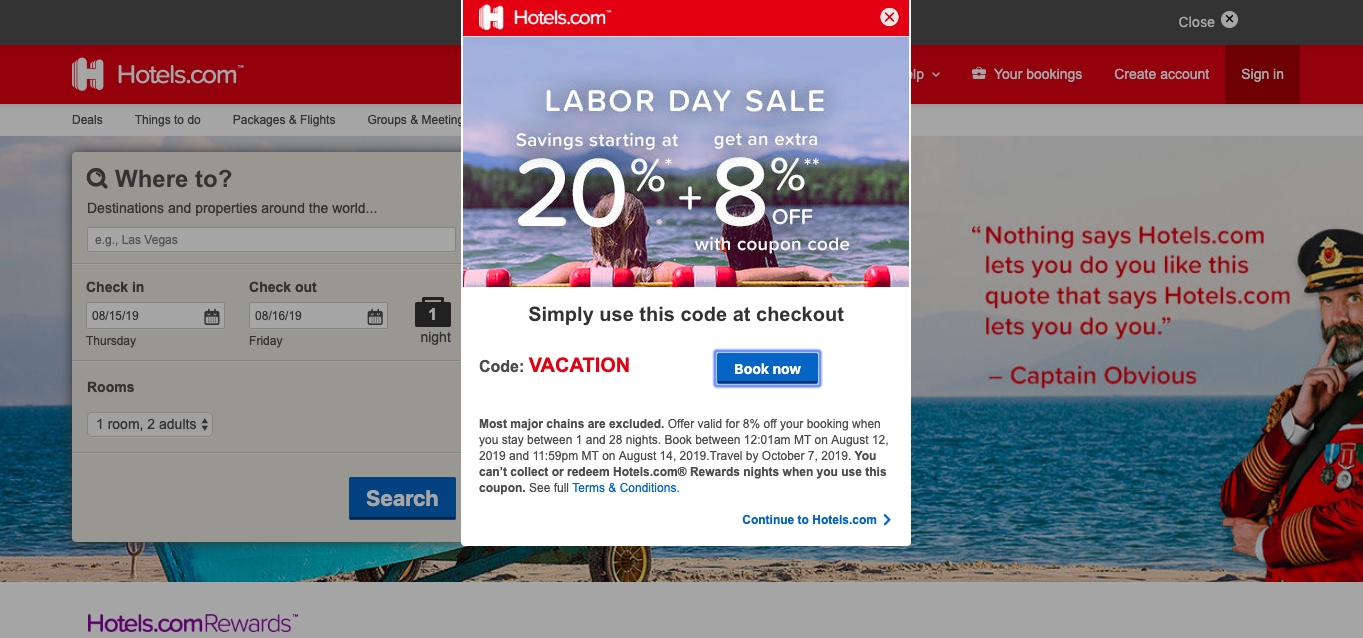This image, sourced from Hotels.com, features a promotional pop-up for a Labor Day Sale. The upper section of the pop-up includes a red bar with an "H" designed to resemble a building, alongside a clickable "X" to close the notification. The background of the webpage is subtly visible in a lighter gray, emphasizing the pop-up's content.

The central focus of the pop-up is a picturesque scene of two individuals gazing out over a serene lake with majestic mountains in the background. Above this scenic image, bold text announces "Labor Day Sale," highlighting savings starting at 20%, with an additional 8% off using a specific coupon code.

The coupon code "VACATION" is prominently displayed in red, capital letters. Below this, a blue "Book Now" button with white text invites users to take action. The bottom section of the pop-up contains detailed promotional information, encouraging users to take advantage of the special offer.